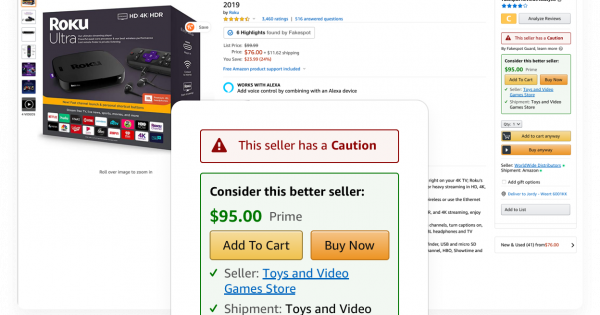**Amazon Product Page for Roku Ultra HD 4K HDR - 2019 Model**

The displayed Amazon product page features the 2019 Roku Ultra HD 4K HDR streaming device. Even though the top portion of the page is cut off, it's clear that this is an Amazon listing. The product boasts an impressive 4.5-star rating from approximately 3,400 reviews. The details become blurry under the resolution specifications, and a prominent pop-up obscures some parts of the page.

**Pop-Up Alert and Offers:**

There's an alert in a light red rectangle with bold red text cautioning potential buyers about the current seller. The pop-up recommends considering another seller offering the product for $95 with Prime shipping, encouraging users to "Add to cart" or "Buy now." This alert is displayed from a seller named "Toys and Video Game Store," with a light green box indicating their shipping policies.

Despite the warning, the original seller lists the Roku Ultra at a price of $76, with an unclear shipping cost that could either be $11.62 or possibly $71.62 due to the illegibility.

**Product Description and Visibility:**

On the right-hand side of the page, another similar pop-up appears reiterating the $95 Prime offer, complete with a warning label overlapping cart and purchase options. Despite these interruptions, the product remains identifiable as the Roku Ultra HD 4K HDR, distinguished as a high-quality streaming choice for consumers.